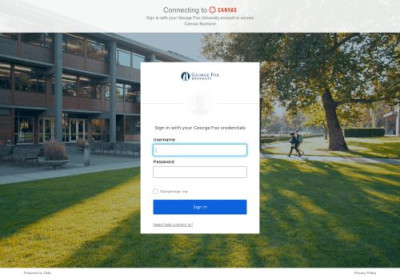In this image, prominently framed by a top banner, we observe a light gray bar extending from left to right. The left segment of this bar features a slightly darker gray section, which contains the text "Connecting to CA and Campuses" in a white font. Beneath this bar, there is a white strip with some blurred text, which is somewhat visible. The central focus is a pop-up window that overlays a scenic backdrop of what appears to be a school campus. On the left side of this backdrop, there is a brick building, partially obscured but distinctly recognizable. Below, a well-maintained grassy area stretches across the bottom of the image, where two students are seen walking towards the building, suggesting a lively and active campus environment.